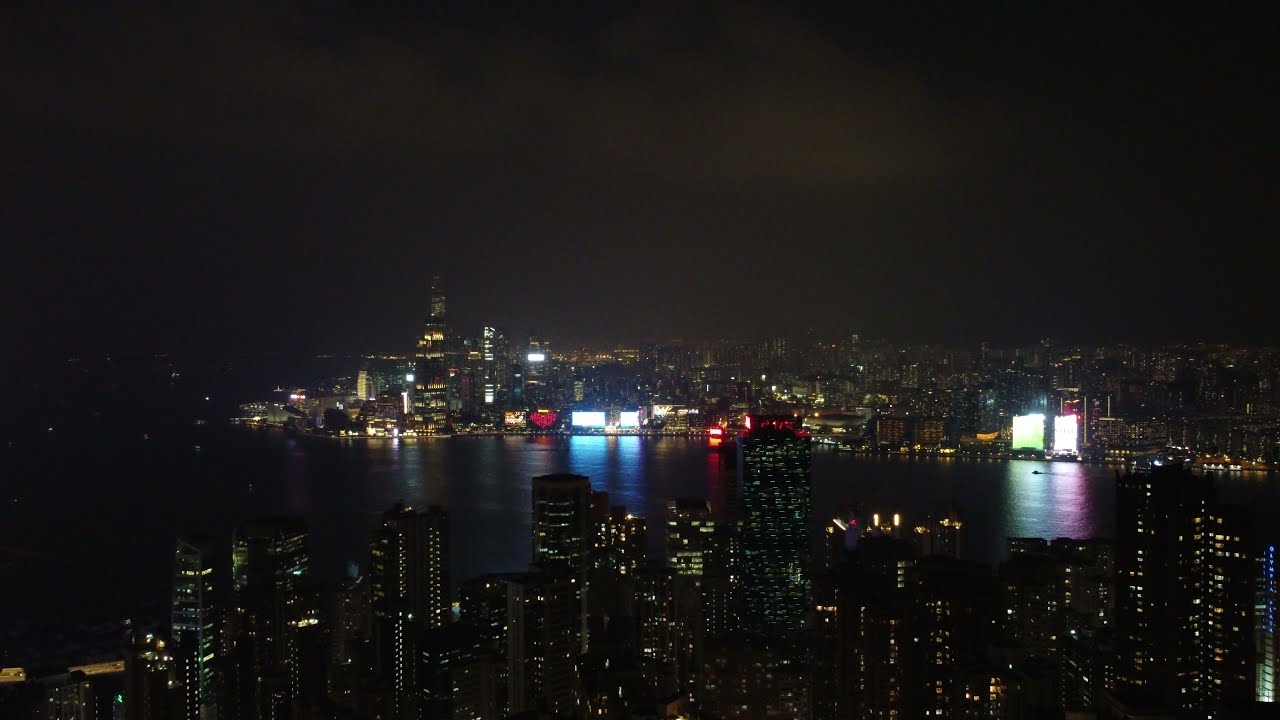The night-time image captures a sprawling metropolis illuminated under a dark sky dotted with distant white clouds. Taken from a high vantage point, the city is nestled along a large, dark body of water that could either be a river or a lake, with the lights from numerous buildings reflecting vividly off its surface. Prominent in the image is a bridge spanning the waterfront, flanked by boats. The skyline is lined with skyscrapers of various sizes, densely packed on both sides of the water, forming a U-shape. Particularly striking are several tall buildings on the right side of the water, their white lights mirroring on the dark water below. Notable among the structures is what appears to be a silhouette of a tall, possibly church-like building on the left-hand side. The waterfront buildings are adorned with bright, colorful lights in hues of red, white, and blue, adding to the vibrancy of the cityscape.